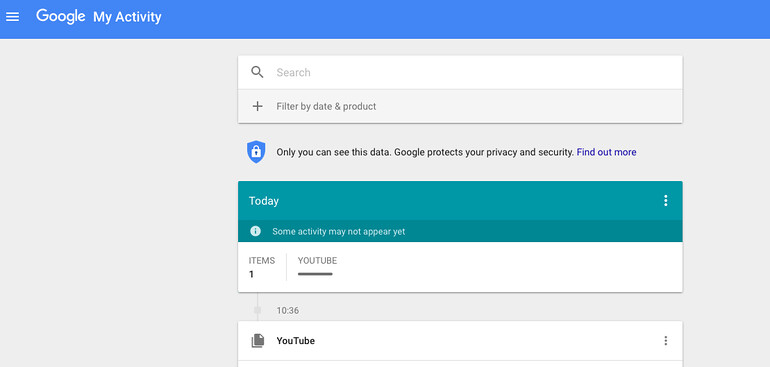This image shows a computer screen displaying a Google My Activity page. The background is a whitish rectangle, with a blue border at the top. On the top left, there is a menu icon consisting of three short white lines stacked vertically in a square. Next to the menu icon, "Google" is written, followed by "My Activity."

In the center of the screen, there is a long white search box with shadowy text that says "Search," accompanied by a magnifying glass icon. Beneath this search box, there is a plus sign with the text "Filter by date & product."

Further down, there is a blue shield with a lock symbol beside the message, "Only you can see this data. Google protects your privacy and security," accompanied by a clickable link that says "Find out more."

A long teal rectangle with the text "Today" in white is shown next, with three white dots on the upper right corner. An information icon—a white circle with a lowercase "i" in italics inside—states, "Some activity may not appear yet."

Below this, there is a chart heading showing "Items," listing one item underneath. The entry labeled "YouTube" indicates an activity timestamped at 10:36. The entry has a small icon resembling sheets of paper, similar to a PDF file icon, followed by the text "YouTube" and another set of three stacked dots for more options. This entry likely represents a YouTube video watched at 10:36.